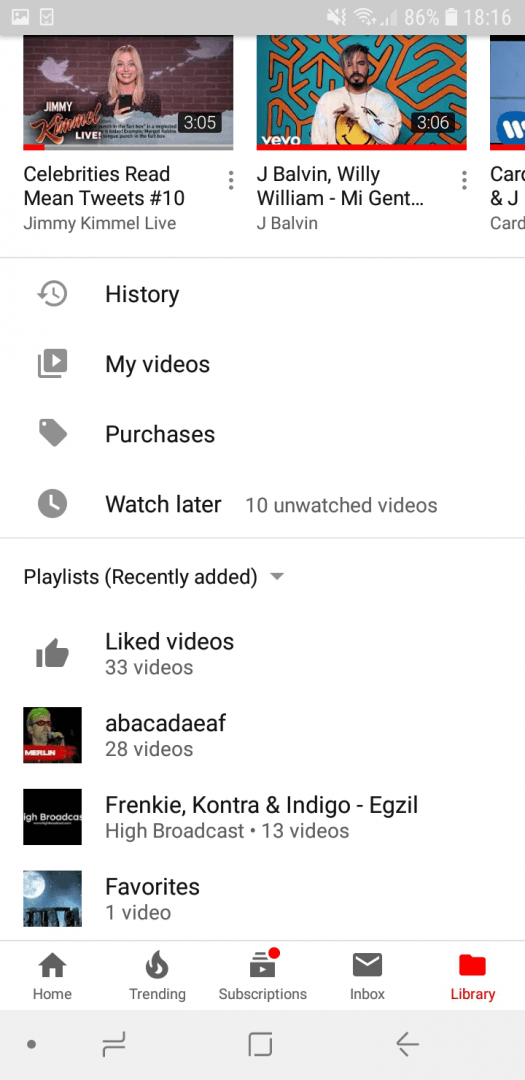The image displayed on the screen portrays a vertically oriented cell phone showcasing a YouTube interface. The screen reveals two nearly full video thumbnails and a partial one on the right. The first thumbnail features a blonde woman with the title "Celebrities Read Mean Tweets #10" from Jimmy Kimmel Live. The second thumbnail belongs to VEVO, displaying "J Balvin, Willy William - Mi Gente" by J Balvin. The partial video on the right is largely obscured, showing only a few indistinguishable letters.

Below these thumbnails, the interface lists several categories: "History," "My Videos," "Purchases," and "Watch Later," which indicates having 10 unwatched items. Further down, a dropdown menu under "Playlists" shows "Recently Added" as the current selection. It also lists "Liked Videos" containing 33 videos, followed by an entry labeled "ABA ACADAEAF," and two additional unspecified entries beneath that.